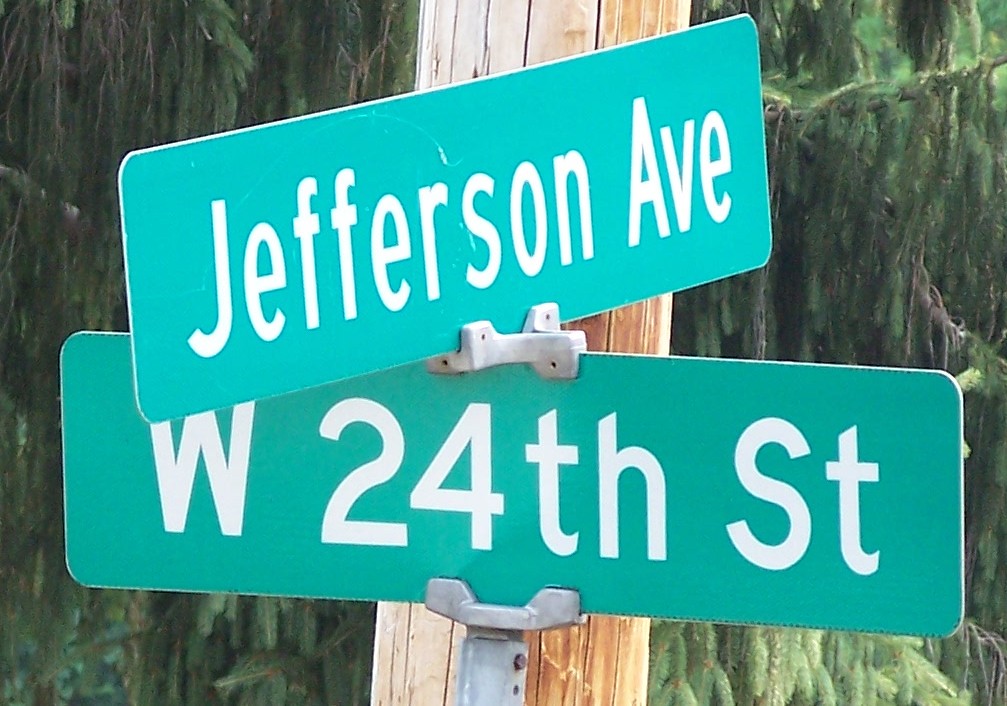A close-up image features two intersecting street signs prominently displayed. A gray metal pole emerges from the bottom of the frame, supporting the signs with sturdy gray brackets. The first sign, positioned more prominently, is a green rectangular placard with bold white lettering that reads "W 24TH ST," indicating West 24th Street. Adjacent to it, a second green sign is attached at a slightly different angle, bearing the inscription "JEFFERSON AVE" in similar white letters. In the background, a light-colored tan utility pole, possibly for telephone or power lines, rises vertically. Further behind, a lush, green tree with drooping branches reminiscent of pine needles, completes the scene, adding a touch of natural greenery to the urban setting.